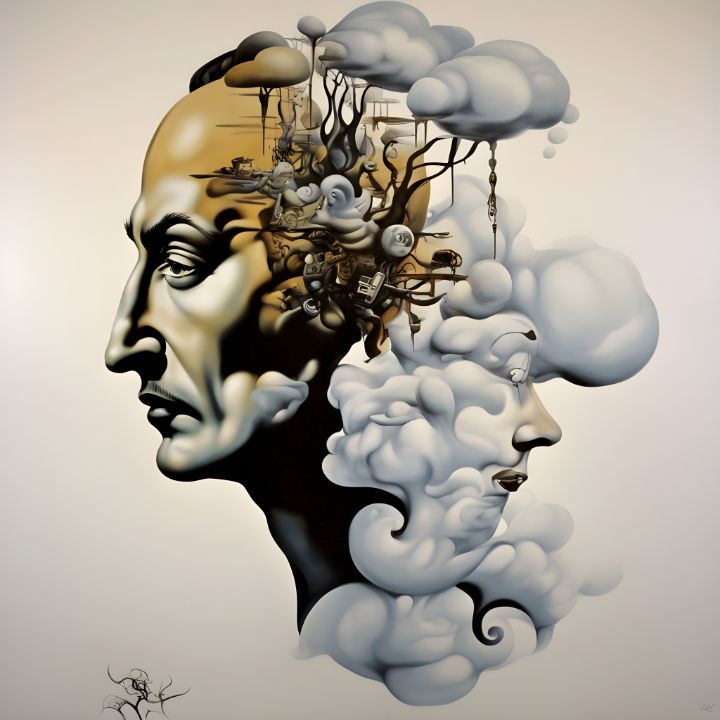This abstract surrealist painting features the contrasting profiles of two faces set against a plain white background. The primary face on the left, portrayed in shades of bronze, gray, and black, depicts a solemn, bald-headed man facing left with distinct features including a long nose, small mustache, and sad, inset eyes. His facial expression is stern and contemplative. Emerging from the top of his head is a vivid scene of turmoil, including mechanical items, an abstract stylized tree with branches replaced by clouds, and various other objects such as an old camera, radio, and animal shapes.

In contrast, the secondary face on the right, appearing to be made of clouds with a wispily rendered form, faces right. This face, which seems more feminine, is less defined with white eyes, thin black eyebrows, and lips that appear to be adorned with lipstick. It is constructed of cloud-like billowy material and seemingly melds into the background. This head also connects to the abstract, chaotic mix of cloud and tree imagery, linking both figures through their shared cerebral landscape.

Overall, the artwork represents a complex interplay of thoughts and emotions, visualized through the contrasting materials and expressions of the two faces, and the surreal, dreamlike elements encased within and around them.